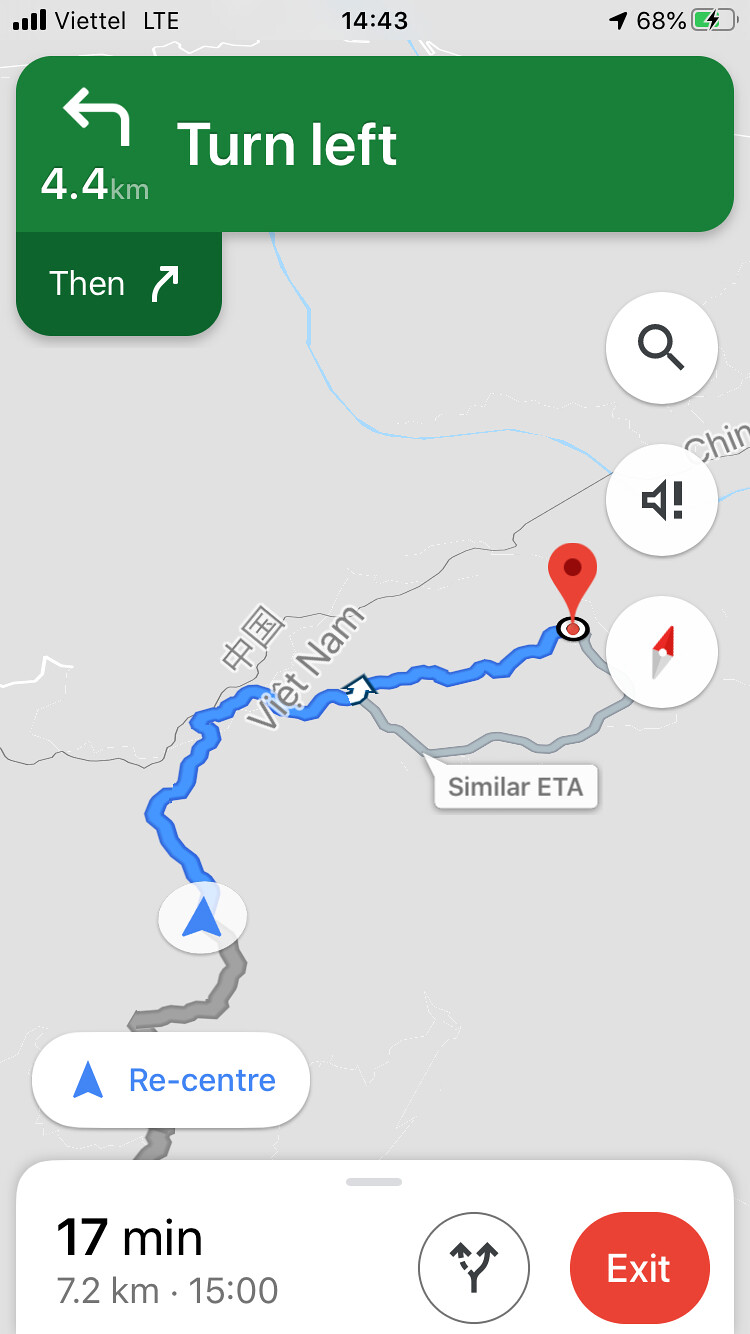The image is a screenshot of driving directions on a cell phone, displaying a route in Vietnam. The map, similar to Google Maps, plots a journey of 7.2 kilometers, estimated to take 17 minutes. The driving instructions note an upcoming left turn in 4.4 kilometers, followed by a right turn. The map appears light gray with the outlined route in blue, culminating in an upside-down red teardrop representing the destination.

Key details include a timestamp of 14:43 and a battery level of 68% on the top right, with the cell service provided by Viettel. Prominently, "Vietnam" is labeled on the map, with "China" visible to the far right. At the bottom, a white rounded rectangle provides travel details—'17 minutes 7.2 km'—alongside a white circle with a blue arrow pointing up, and a red button labeled 'exit'. The visual interface includes a green rectangle at the top instructing a left turn with a left-arrow icon, followed by an additional smaller green rectangle with a right-arrow icon. There is also a white text box at the lower left saying 're-center', emphasizing navigation options.